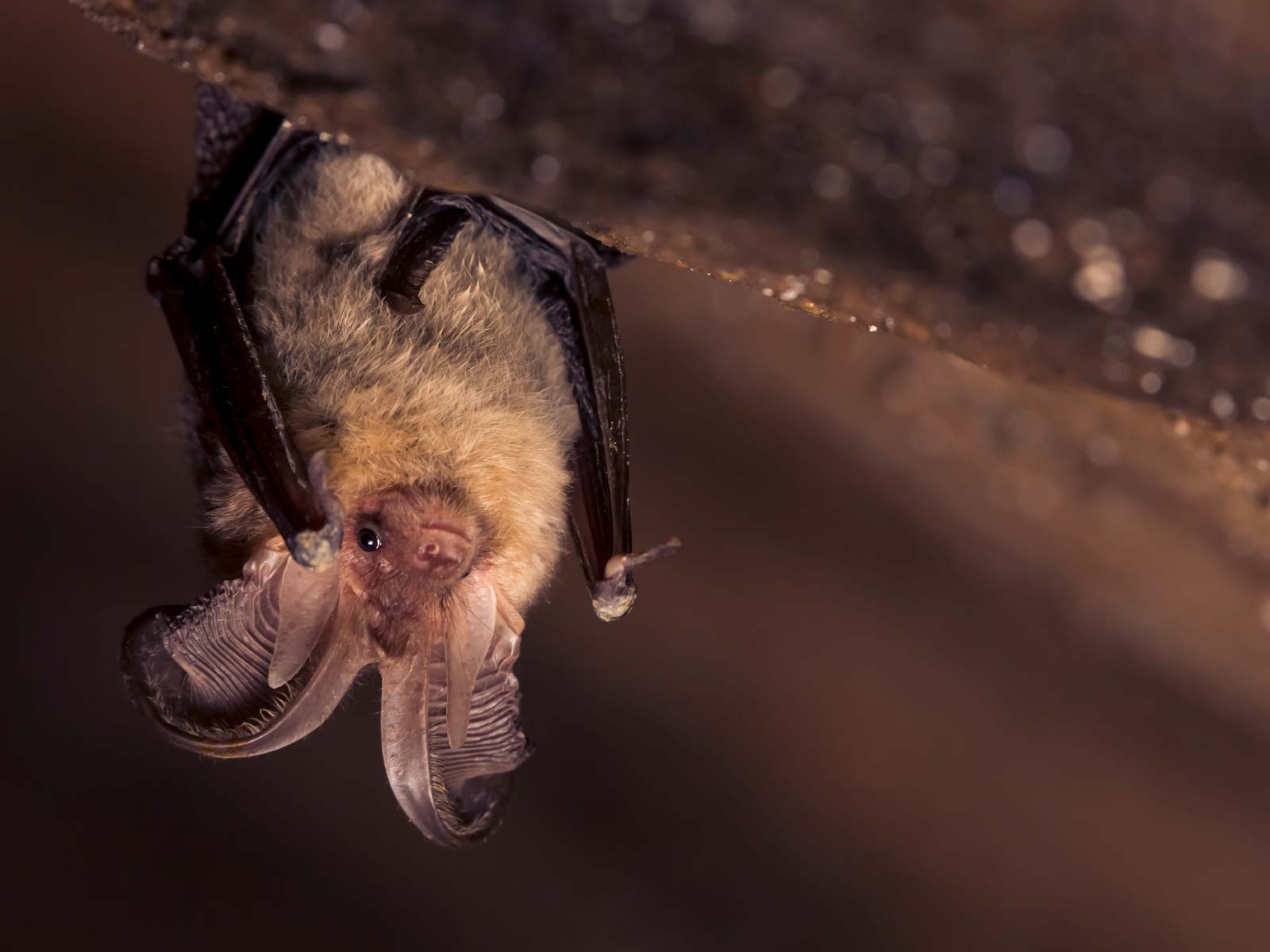The image is a high-quality, close-up photograph of a small bat hanging upside down inside a dark, moist cave. The bat, roughly the size of a small person's fist, is situated on the upper left side of the image, clinging to a dark brown surface that features some water droplets. The bat's wings are folded behind its ears, which are notably large relative to its head. Its fur is primarily brown with a light-colored patch around its face that contrasts with its black eyes. The bat's eyes are open, staring directly towards the camera, indicating it is not sleeping. The natural lighting in the cave illuminates the bat, creating a clear and bright setting despite the generally dark surroundings. No other bats, people, numbers, or text are present in the image.